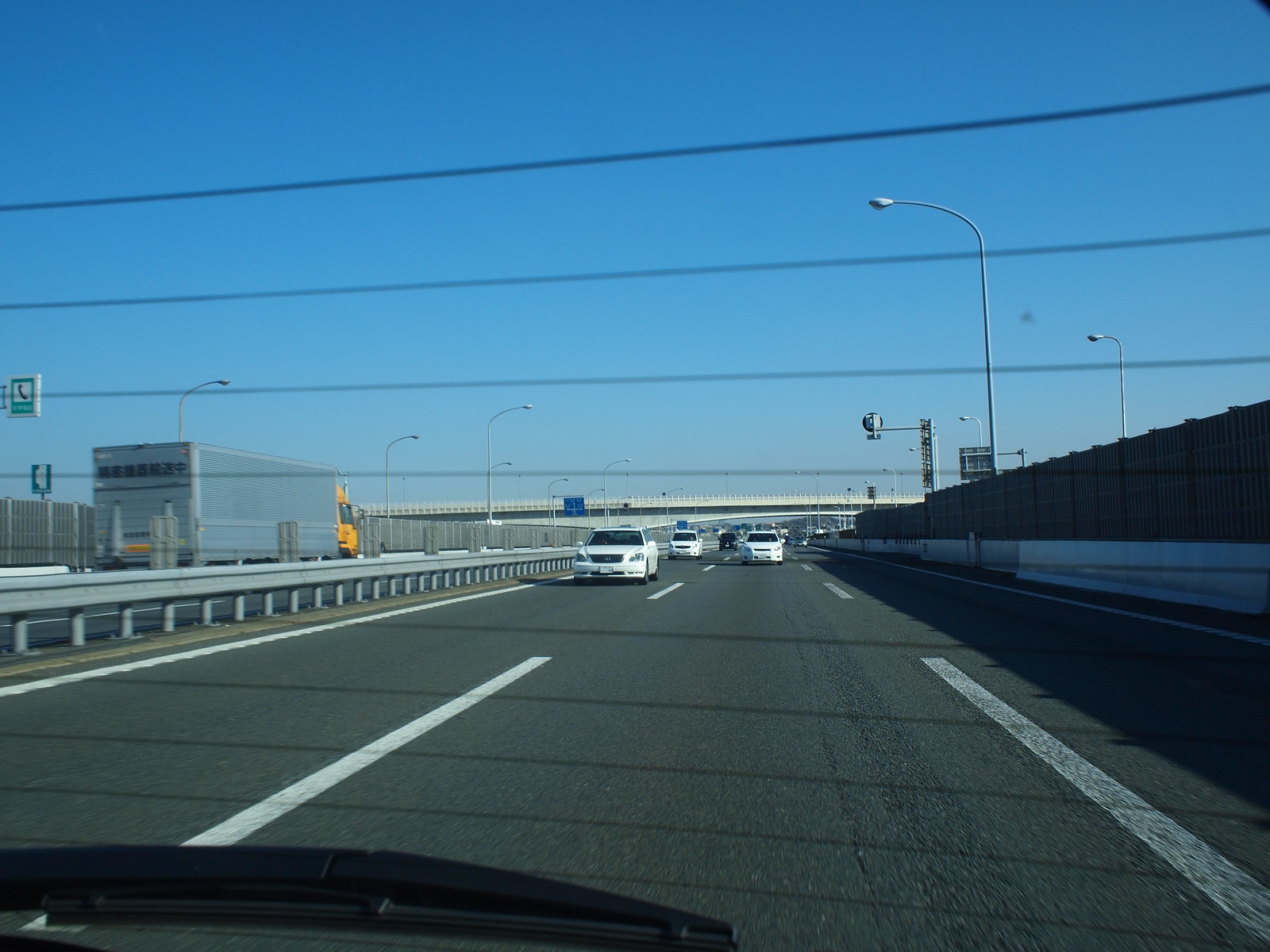The image captures a view through the back window of a car traveling on a three-lane highway, framed by several horizontal black lines, likely on the glass. The highway stretches ahead, featuring white dashed lines dividing the lanes and bordered by solid white lines. Several vehicles are visible: two white sedans closely following each other in the left lane, another white sedan in the right lane, and a black vehicle further back. To the left, an 18-wheeler truck with a yellow cab and a silver trailer adorned with black Chinese characters is heading in the opposite direction, separated by a steel guardrail. The sky transitions from dark blue at the top to lighter blue towards the horizon, where highway lights and signs with telephones are visible. Tall, gray or silver walls and fencing line both sides of the road. A windshield wiper is located at the bottom left corner of the car's rear window, adding to the detailed observation of the scene.